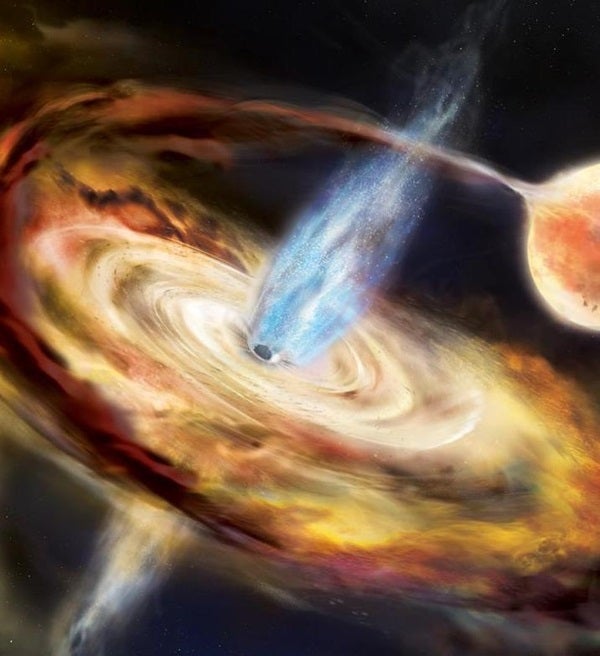This image is a detailed artistic render depicting a dramatic cosmic event in outer space, featuring a black hole consuming a nearby star. At the center, a disk of swirling gas brightens intensely as it spirals into the black hole. This gas originates from a stream visibly extending from a star located on the right side of the image, arcing towards the left before being pulled into the black hole. Emphasis is placed on the luminous orange and white center of the black hole, enveloped by a contrastingly dark, black background. Streams of gas, possibly representing Hawking radiation, are shown ejecting from both poles of the black hole - a vivid blue jet being particularly prominent on the upper side. The entire scene, with its starkly colorful, highly detailed elements against the dark void of space, creates a visually arresting and scientifically intriguing depiction of a celestial phenomenon.